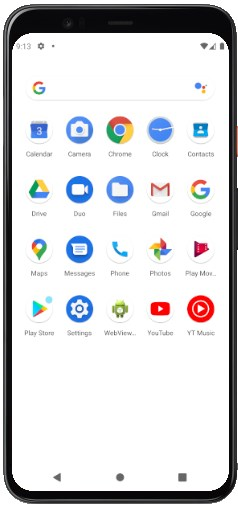The image is an illustration of a smartphone displaying a realistic-looking screenshot. The smartphone has black borders at the top, with slightly rounded corners that reflect light, adding a touch of gray. The screen itself is white, showing the time as 9:13, though it does not specify whether it’s AM or PM. On the right side of the screen, there are three status icons: Wi-Fi, wireless signal strength, and a fully charged battery.

At the very top of the screen is the Google search box, outlined as a rounded rectangle featuring the colorful Google "G" logo and the Google Assistant icon, depicted as a blue dot accompanied by smaller red and yellow dots.

Below the search box are neatly arranged app icons, all from Google, displayed in a grid of four rows and five columns, making up 20 icons in total. The visible apps include Calendar, Camera, Chrome, Google Drive, Google Duo, Gmail, the main Google app, Maps, Play Store, YouTube, among others.

Finally, at the bottom of the screen, there is a small blank space followed by a central navigation bar featuring three icons: a gray circle in the center for the home button, a left-pointing triangle on the left for the back button, and a small square on the right for the recent apps button.